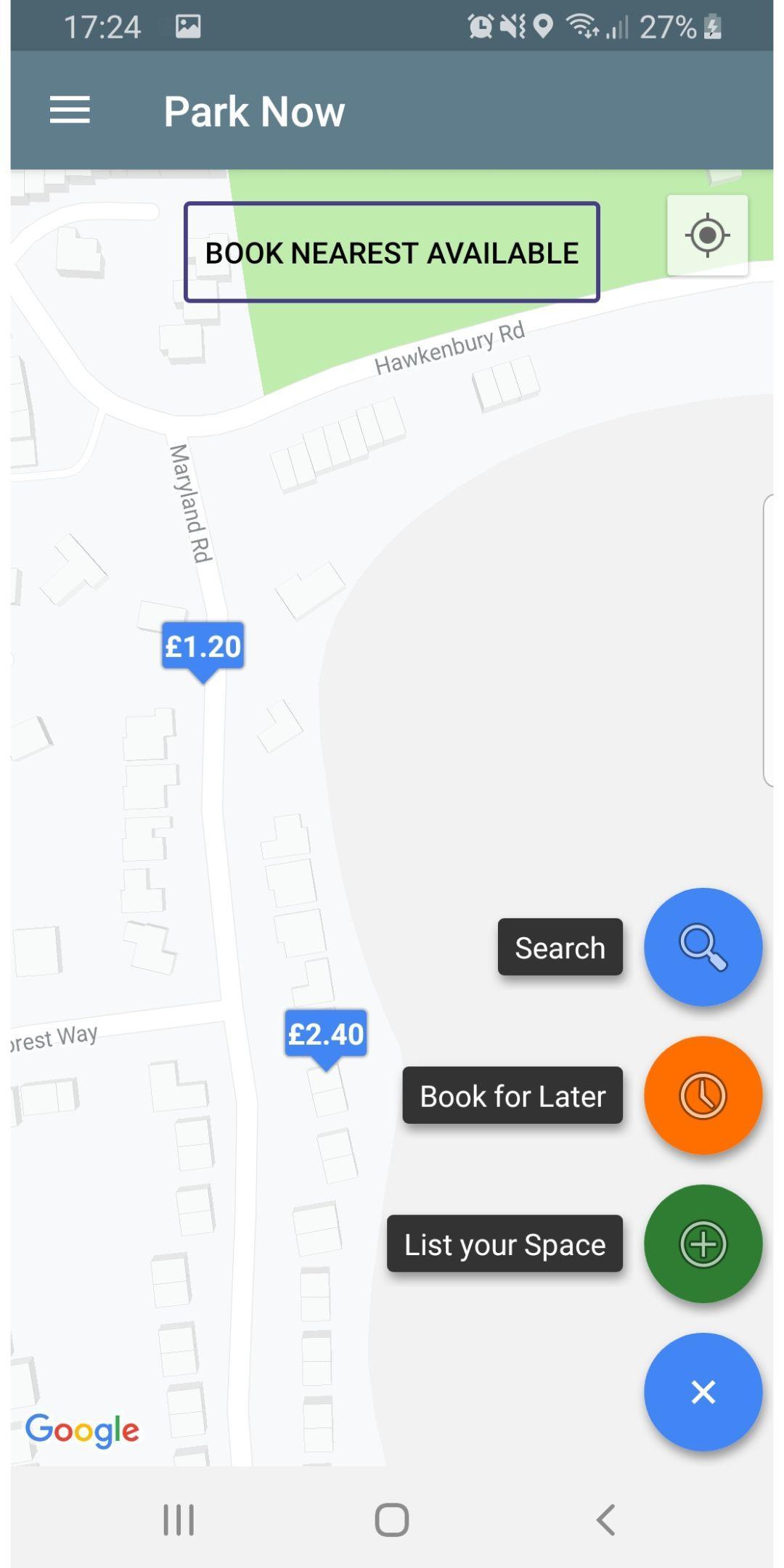The image depicts a user interface on a mobile device, likely a phone but possibly a tablet, showing a parking application map from Google. The top of the screen displays the time "17:24" in white letters against a dark gray background, along with various status icons, such as the phone signal bars (showing 2 bars), the battery level at 27%, and an icon of a person. Below this, a thicker gray bar features the text "Park Now" in white, with three horizontal lines indicating a menu for more options.

The map prominently displays streets named Hockenberry Road and Maryland Road, which converge at an intersection with Forrest Way. The map also highlights parking options with prices listed in British pounds, such as £1.20 and £2.40, suggesting it is set in the UK. There is a compass icon for orientation and a button labeled "Book Nearest Available" in a black box.

Additional features on the interface include a search bar with an adjacent icon, a "Book for Later" option accompanied by a clock icon, and a "List Your Space" button with a green plus sign in a black box. An X icon is also present to close the interface. In the bottom left-hand corner, the word "Google" confirms the map's association with Google services.